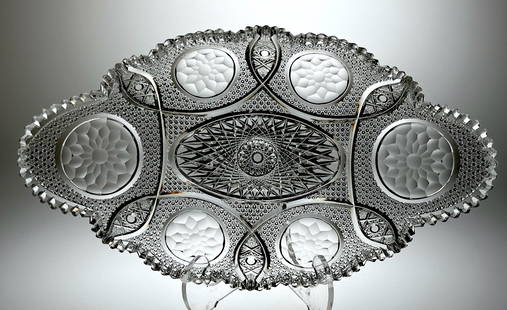This black-and-white photograph features an intricate cylindrical piece of glass, horizontally positioned on a clear Lucite stand. The glass, possibly part of an elaborate serving tray or a piece of decorative jewelry, is adorned with an ornate border of small round bumps, giving it a textured look. Along its length are various circular elements arranged in a precise pattern: two circles at the top, two at the bottom, one central cylindrical circle, and one on each side. Some circles are light in color, while others are darker, all embellished with floral designs. Additionally, swirling lines and what appears to be metal loops or draped elements interlace these circles, adding to the detailed and decorative nature of the piece.